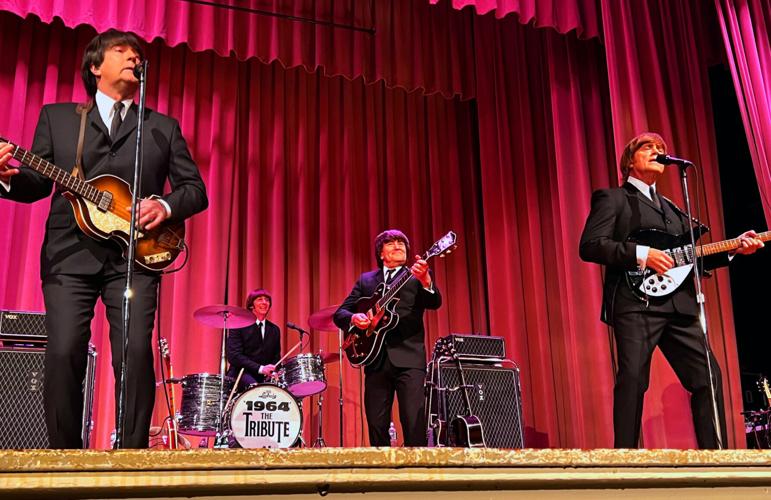The image captures a dynamic moment of a Beatles tribute band performing on stage. The four band members are wearing dark suits with white collars and black ties, evoking the classic Beatles look, complete with the iconic bowl haircuts. They are positioned in front of a luxurious maroon curtain that forms the stage backdrop. The drummer, who sports the same distinctive haircut, sits at his drum set, which prominently features "1964 The Tribute" along with a logo reminiscent of The Beatles. In the foreground, three members stand, each holding a guitar and singing into microphones. One guitarist is positioned next to a black speaker on the left of the stage, while the other two flank the stage's front, all immersed in their performance under bright stage lights. The photograph appears to be taken from the audience's perspective, capturing the energy and homage of this dedicated cover band.